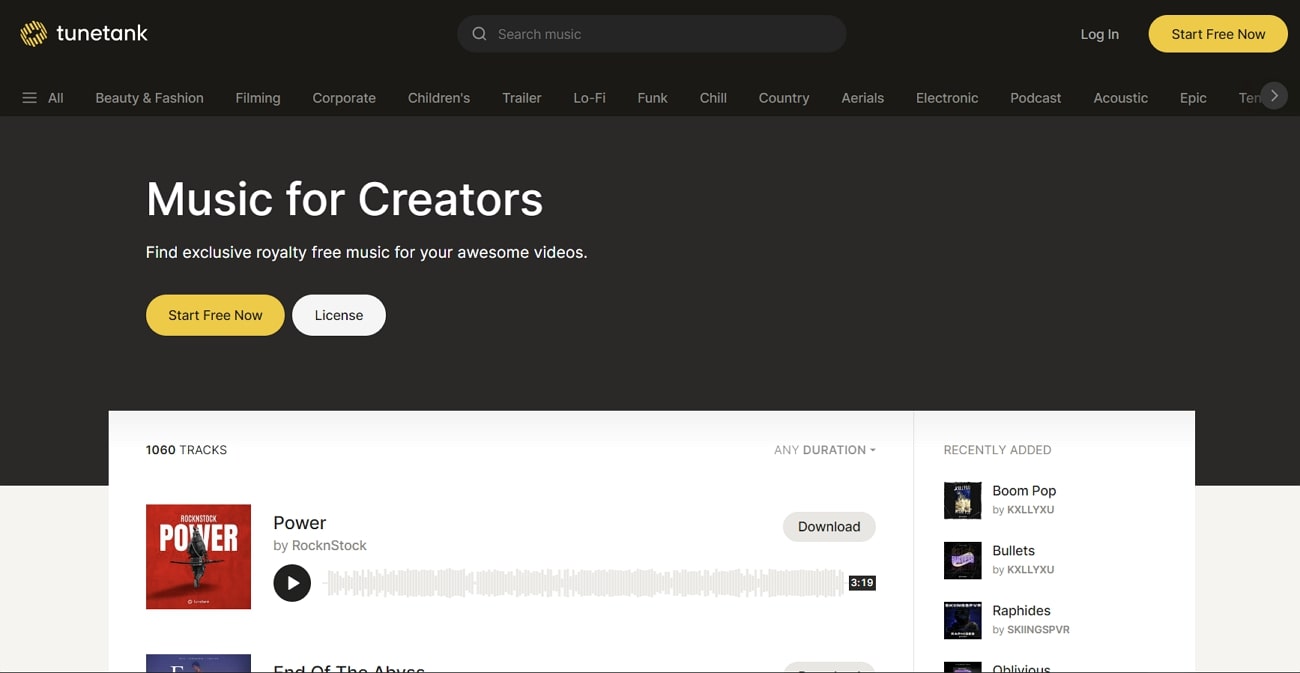A desktop screenshot of the Toontank music website is displayed. At the top of the page, a dark grey header features a yellow circular logo with "Toontank" in white text on the left side. In the center of the header, a light grey search bar is positioned. On the right side, there is a login button and a prominent yellow button with "Start Free Now" written in black. Below the main header are several light grey text buttons signifying different music genres, including an "All" button, a "Menu" button, and an arrow button.

Just beneath this, against a lighter grey background, there is bold white text that reads "Music for Creators." Directly underneath, in smaller white text, is a centered tagline: "Find Exclusive Royalty-Free Music for Your Awesome Videos." To the left side, a yellow button with "Start Free Now" in black is situated, alongside a white button labeled "Licence." The right side of this section contains empty grey space.

Below these elements, the webpage's background transitions to white, and across both the grey and white portions, an image displays a collection of music tracks. On the left, a track titled "Power" with a red cover includes a play button, a timer showing 3 minutes and 19 seconds, and a download button. On the right side, a "Recently Added" list is showcased, featuring four songs: "Bomb Boom Pop," "Bullets," "Raphides," and "Oblivious," each with distinct cover art and titles.